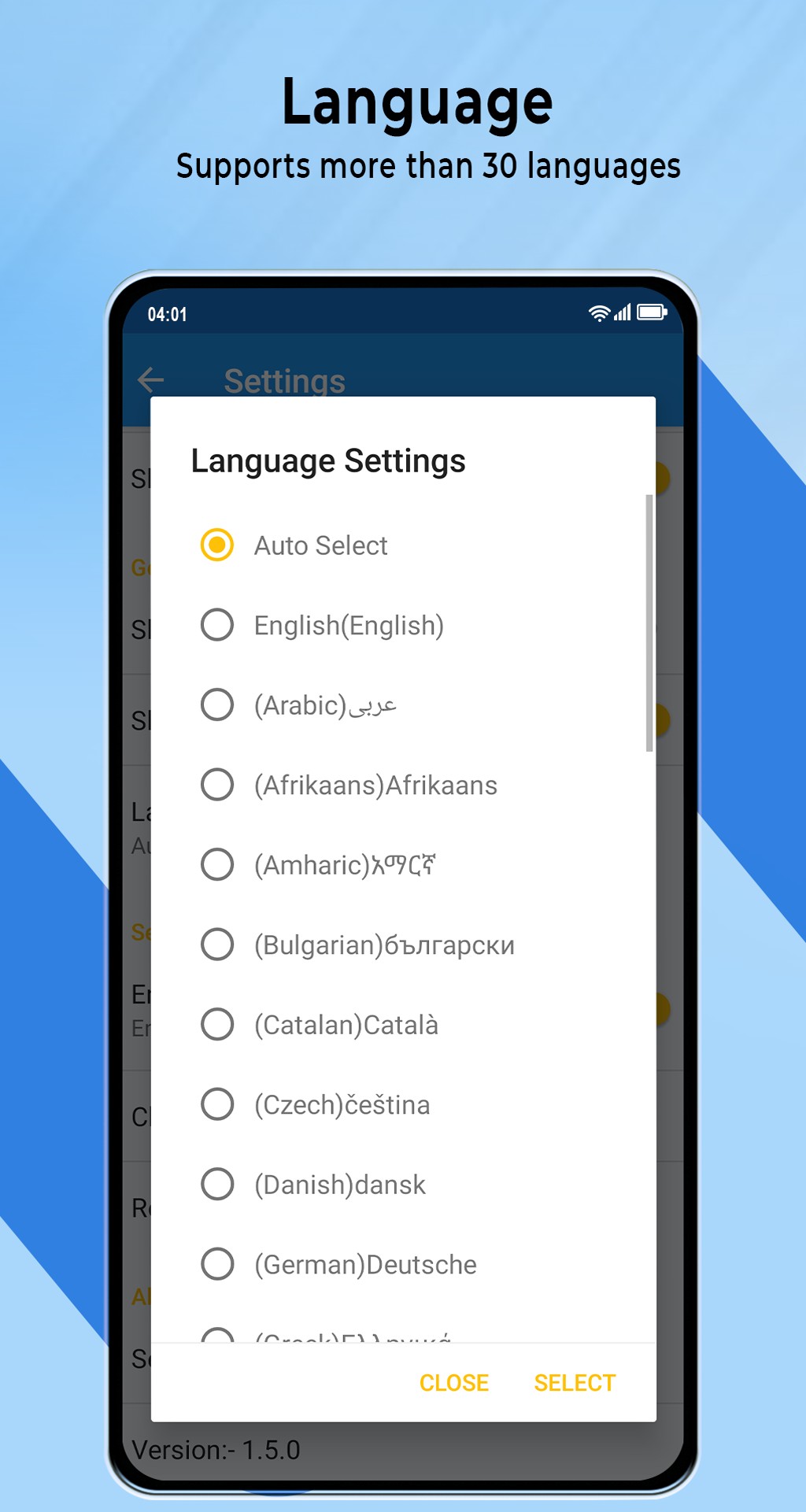The image is a detailed screenshot of a cell phone against a dual-tone light and dark blue background. The cell phone, which has a black outline around its screen and a possible gray top edge, displays the following details:

1. **Interface Elements:**
   - **Time:** It is 4:01.
   - **Status Indicators:** To the right, in white, are icons for the WiFi signal, wireless signal, and battery level.

2. **Foreground Elements:**
   - There is a prominent white box overlaying the background information on the screen. This box is labeled "Language Settings" in black text.

3. **Language Selection Menu:**
   - The box contains vertically arranged white circles, each outlined in black, alongside language options. These options read as follows:
     - Auto-select (selected, indicated by a white dot with a dark yellow center and ringed in yellow)
     - English (in brackets)
     - Arabic (in brackets, followed by Arabic script)
     - Afrikaans (in brackets, repeated again as Afrikaans)
     - Amharic (in brackets, followed by Amharic script)
     - Bulgarian (in brackets, followed by Cyrillic script)
     - Catalan (in brackets, noted as "Català" with a tilde over the last 'a')
     - Czech (in brackets, as "Čeština" with accents over the 'C' and 'e')
     - Danish (in brackets, as "Dansk")
     - German (in brackets, as "Deutsch")

4. **Additional Interface Text:**
   - At the top of the white box, the bold black text reads "Language."
   - Below it, a smaller black font states "supports more than 30 languages."
   - Below the list of languages, there are two buttons labeled "Close" and "Select" in yellow, with a corresponding dark yellow dot for selection marking.

This captures the structure and details of a phone language settings screen, emphasizing the language selection process and the layout of various UI elements.